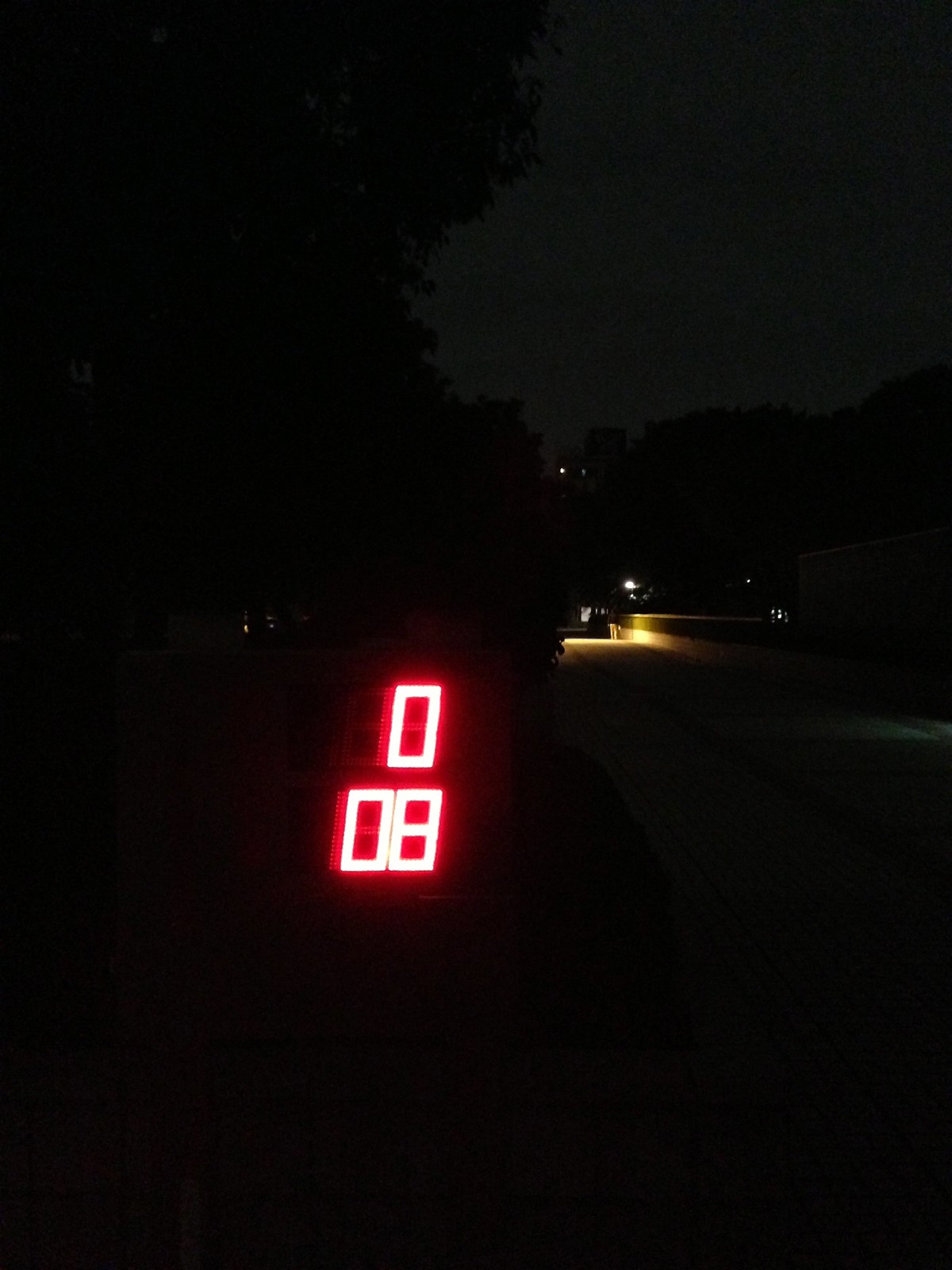In the image, a dark street at night serves as the backdrop for a striking focal point: a set of illuminated numbers glowing in ominous red. At the top of this numeric display is a '0,' with '08' positioned directly beneath it. The specific purpose or reference of these numbers remains unclear, shrouded in mystery. The numerical display is suspended in the pitch-black street, adding a surreal touch to the scene. Behind it, vague silhouettes of darkened trees attempt to pierce through the darkness. Towards the end of the street, a lone source of light attempts to break through the night, casting a dim glow on what appears to be a privacy wall, though it fails to provide any significant illumination.

On the right side of the frame, the faint outline of a square building barely emerges from the shadows. The night sky, devoid of stars, maintains a faint luminescence that subtly outlines the trees in the foreground, giving them a ghostly appearance. Despite these faint glimmers, the picture remains predominantly dark, punctuated only by the eerie red numbers and the diffused, ineffective light at the street's end.